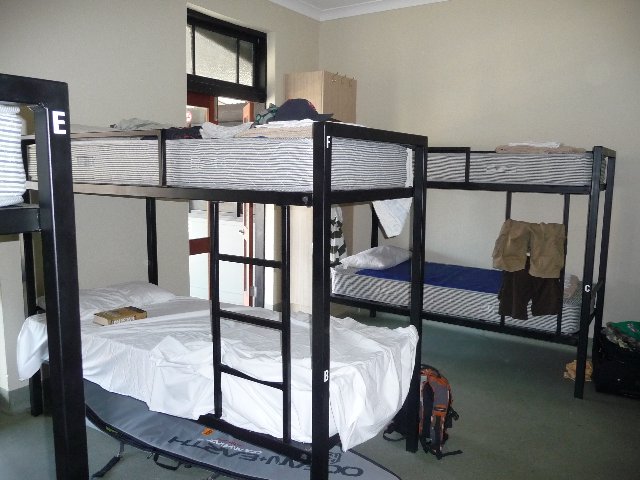The photograph depicts the interior of a simple, functional dormitory room, likely a youth hostel or a transient accommodation. The room features three black metal bunk beds, each with two sleeping units, amounting to six beds in total, all lined against one wall. The mattresses are thick with varying patterns of grey and white stripes—some horizontal, some diagonal. Evidence that the room is often in use by different, temporary occupants includes several mattresses without sheets, suggesting frequent turnover.

Personal items like backpacks, small luggage, and a surfboard in a case are scattered on the floor and beneath the beds, indicating current occupants. Clothes, including men's cargo shorts in tan and olive green, hang off the ends and ladders of the bunk beds. Notably, a book lies near a pillow on the bottom bunk closest to the viewer, enhancing the lived-in atmosphere. The far end of the room features a clothes dresser with hooks above it, and a doorway to the hall is visible to its left. The overall setting emphasizes a transient lifestyle, with minimal personal touches and a focus on functionality.